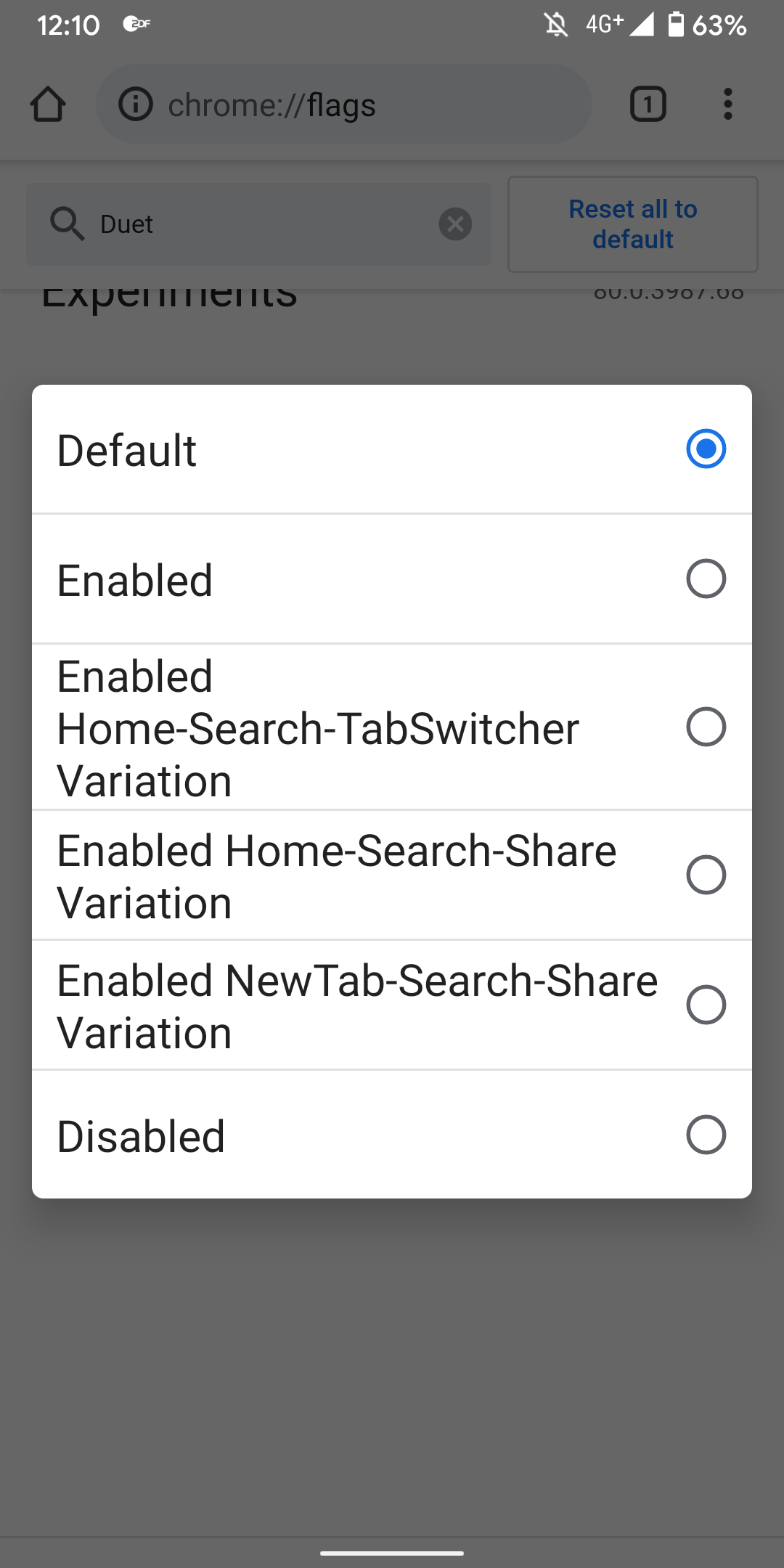The image appears to be a screenshot taken from a mobile device, specifically showing a gray-themed background. Central to the image is a prominent white square featuring a list of options associated with the Chrome browser settings. These options include "Default," "Enabled," "Enabled home search tab switcher variation," "Enabled home search share variation," "Enabled new tab search share variation," and "Disabled." Each option is accompanied by a clickable circle, with the "Default" option currently selected by the user.

In the gray background behind the white square, the Chrome browser options are apparent, particularly the URL "chrome://flags" displayed in the search bar, with the term "duet" entered in the search field. To the right in blue, a clickable option titled "Reset all to default" is visible. Below this is the word "Experiments," partially cut off by the browser's search functionality.

Additional details include the device's status bar at the very top, showing it is 12:10 PM with notifications and sound silenced. The device is connected to a 4G+ cellular network, and the battery is at 63% charge.